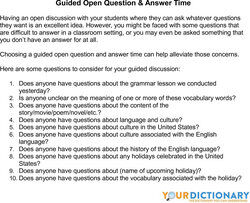The image depicts a text graphic with the title "Your Dictionary" prominently displayed. The word "Your" is written in bold orange letters, while "Dictionary" appears right beside it in striking blue letters, all set against a crisp white background, ensuring maximum readability.

Below the title, there is a comprehensive list of guided questions designed to facilitate an open question-and-answer session with students. The purpose of this session is to encourage an interactive discussion where students feel comfortable asking about any uncertainties they might have. These questions span a broad range of topics, ensuring that various aspects of the students' learning experience are covered:

1. "Does anyone have questions about the grammar lesson we conducted yesterday?"
2. "Is anyone unclear on the meaning of one or more of these vocabulary words?"
3. "Does anyone have questions about the content of this movie, poem, or novel?"
4. "Does anyone have questions about language and culture?"
5. "Does anyone have questions about the culture and the outside world?"
6. "Does anyone have questions about the culture associated with the classroom?"
7. "Does anyone have questions about the history of the language?"
8. "Does anyone have questions about any holidays celebrated in the Odyssey?"
9. "Does anyone have questions about the name of the upcoming holiday?"
10. "Does anyone have questions about the vocabulary associated with the holiday?"

These structured questions are thoughtfully designed to guide the discussion, helping the teacher manage the conversation effectively while ensuring that all students' concerns and queries are addressed comprehensively.